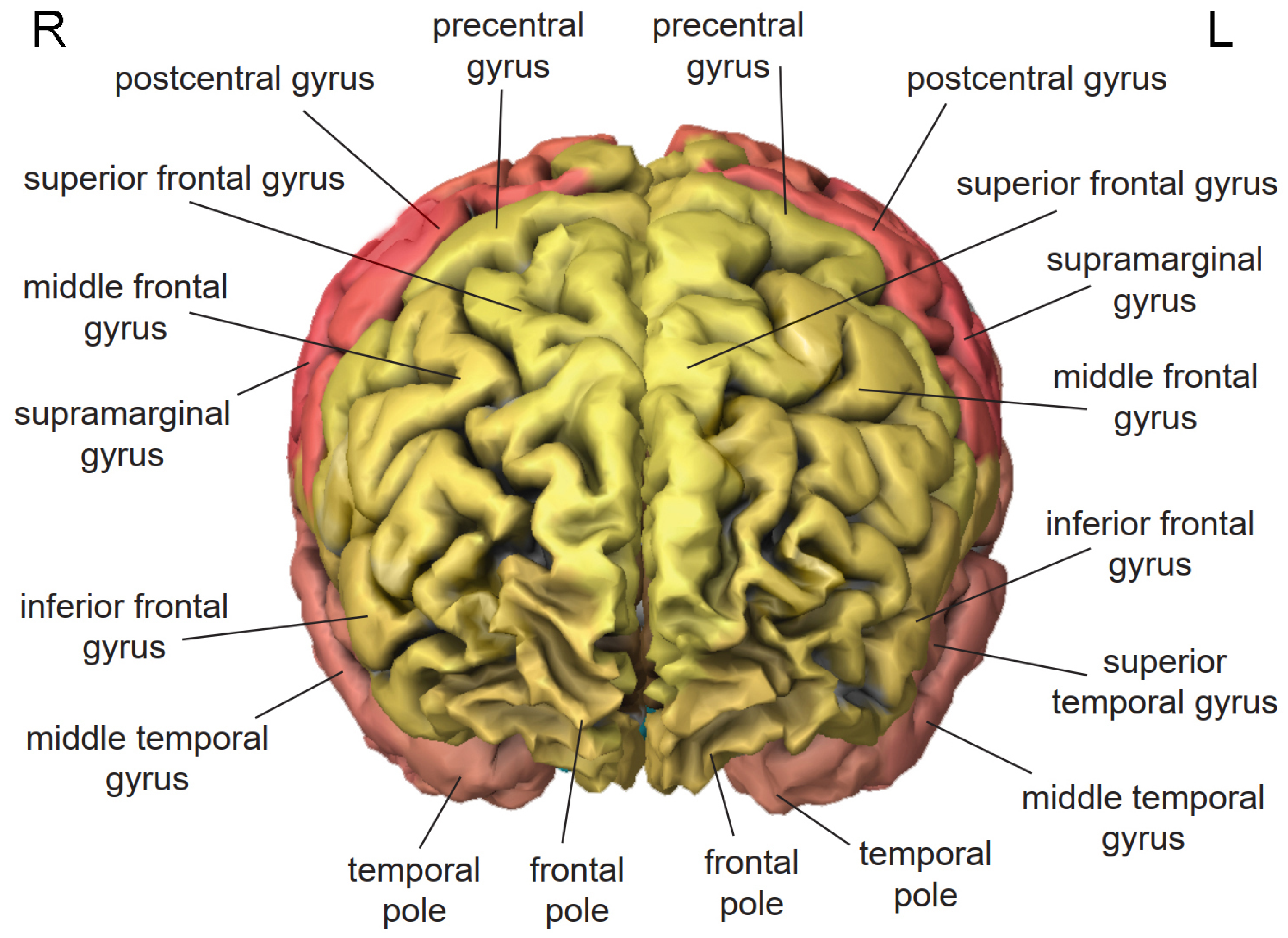This detailed instructional image, presumably from a medical or anatomy textbook, depicts a top-down view of the brain, focusing on its hemispheres. The brain is largely gold in color with a pink outer edge. The background is white, with black type used for labeling. On the top left of the image is a bold "R," and on the top right, a bold "L," indicating the right and left sides of the brain. Various anatomical terms are meticulously labeled around the brain with arrows pointing to corresponding areas. Starting from the top and moving clockwise, the labels include precentral gyrus, postcentral gyrus, superior frontal gyrus, supramarginal gyrus, middle frontal gyrus, inferior frontal gyrus, superior temporal gyrus, middle temporal gyrus, temporal pole, and frontal pole. The labeling is mirrored across both hemispheres, ensuring comprehensive identification of each part.